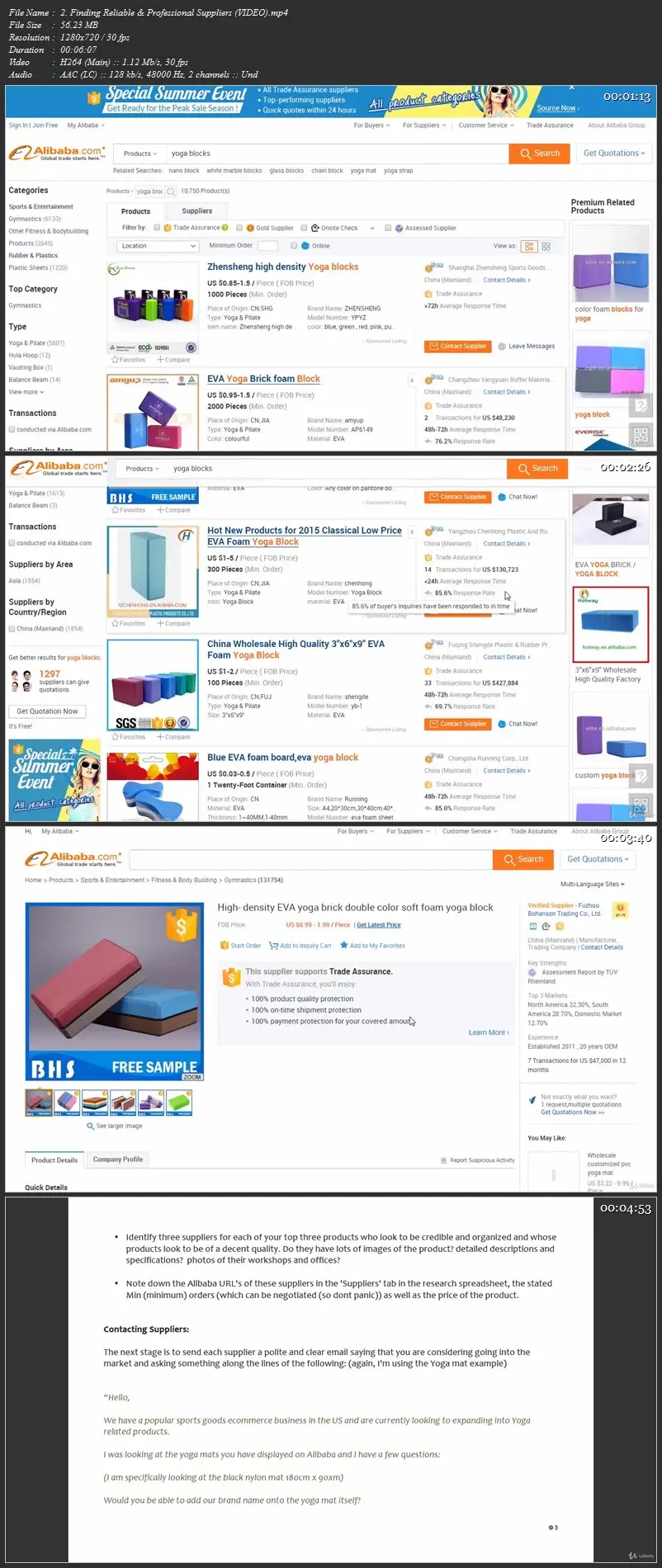The image appears to be a promotional page from a shopping website advertising a "Special Summer Event." At the top of the page, there is a header with small print, which is difficult to read. The header is highlighted by white text on a blue background, announcing the special event, and includes a yellow image of a woman wearing sunglasses. Above this, there is an inscription that is barely visible. 

Prominent at the top is a large black bar filled with white text, providing important navigation and information for the site. Below that, the page transitions to a visually busy layout with a white background. On the left-hand side, there is orange text prominently displayed, alongside a variety of categories listed in black.

The middle section of the page features a "Super Summer Event" theme, with highlighted products, including water bottles. These products are marked by orange boxes at the end of the descriptions, which presumably serve as purchase buttons. Beneath this, there is a colorful assortment of blocks in purple, pink, and blue.

Further down, the layout becomes more structured. A vertical blue box is present in the middle, flanked by smaller boxes in red, purple, blue, and green. Additionally, two images of items that have irregular shapes but are not clearly defined are shown, interspersed with more orange purchase buttons.

The subsequent section is larger and is labeled "BHS," showcasing two items that appear to be yoga blocks or step platforms, likely intended for exercise purposes. These also have purchase options included.

At the very top of the page, there is a search bar for user convenience. Another section follows, characterized purely by text. It contains bullet points and paragraphs, but the text is either too small or too dark to read easily, making the headlines and content unclear.

In summary, this page presents a detailed and vibrant display of items and categories related to a special summer shopping event, with a variety of navigational and purchasing elements aimed at enhancing the user experience.